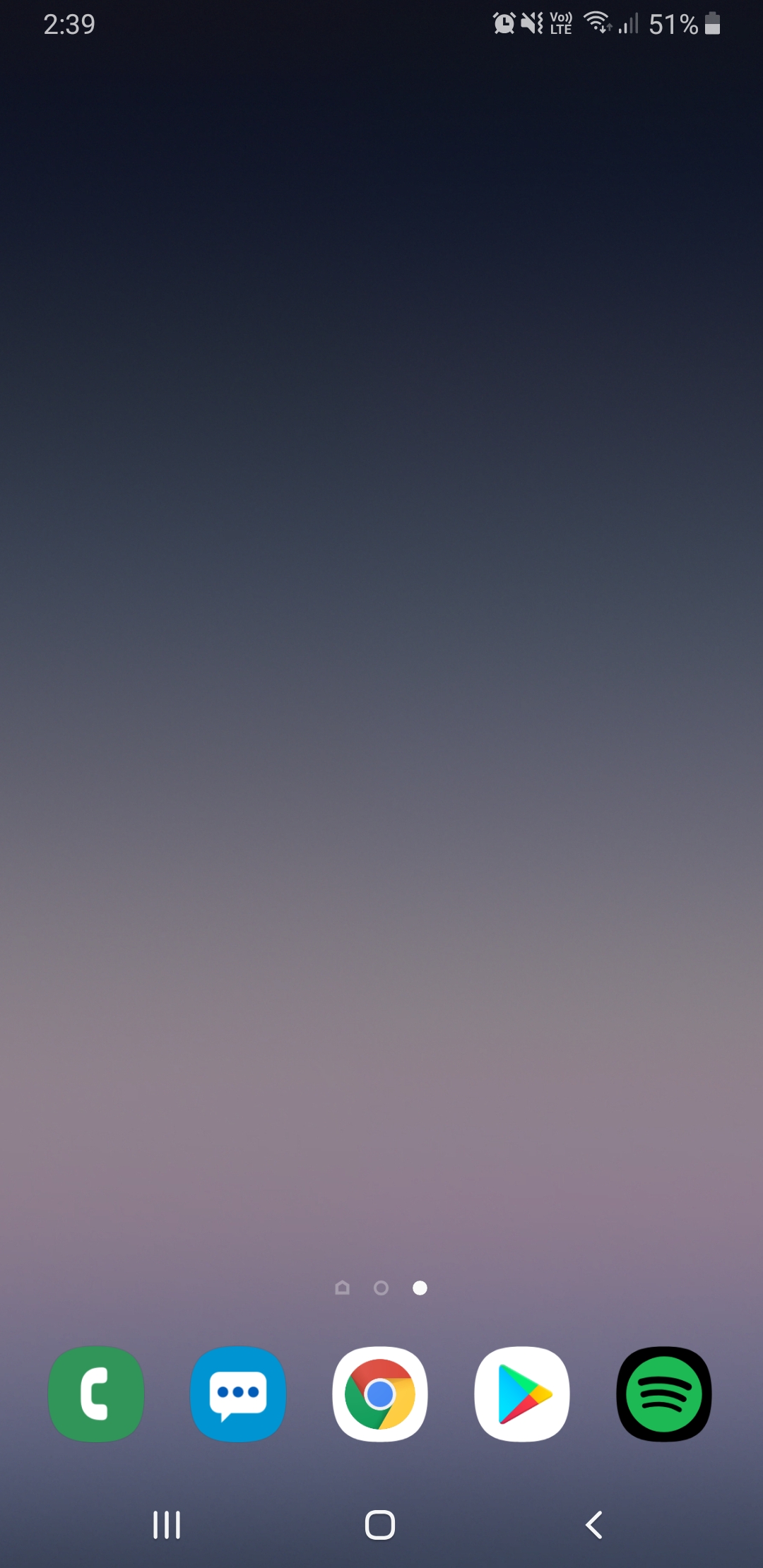The screenshot captures an Android mobile device at 2:39 PM. On the top-right corner, various status icons are visible: a strong signal indicator, a Wi-Fi symbol showing two bars, and a battery icon displaying 51% charge. The screen is on the third page of the home menu, which appears empty and features a gradient background transitioning from black to gray. 

At the bottom of the screen, five primary app icons are lined up: “Phone” on the far left, next to a “Text” messaging app, with the “Google Chrome” browser centrally positioned. To its right, the “Play Store” icon is present, followed by the “Spotify” icon on the far right.

Beneath these icons, the typical Android navigation buttons are displayed – a set of three buttons, including the recent apps button on the far left, a rounded home button in the center, and a back button on the right.